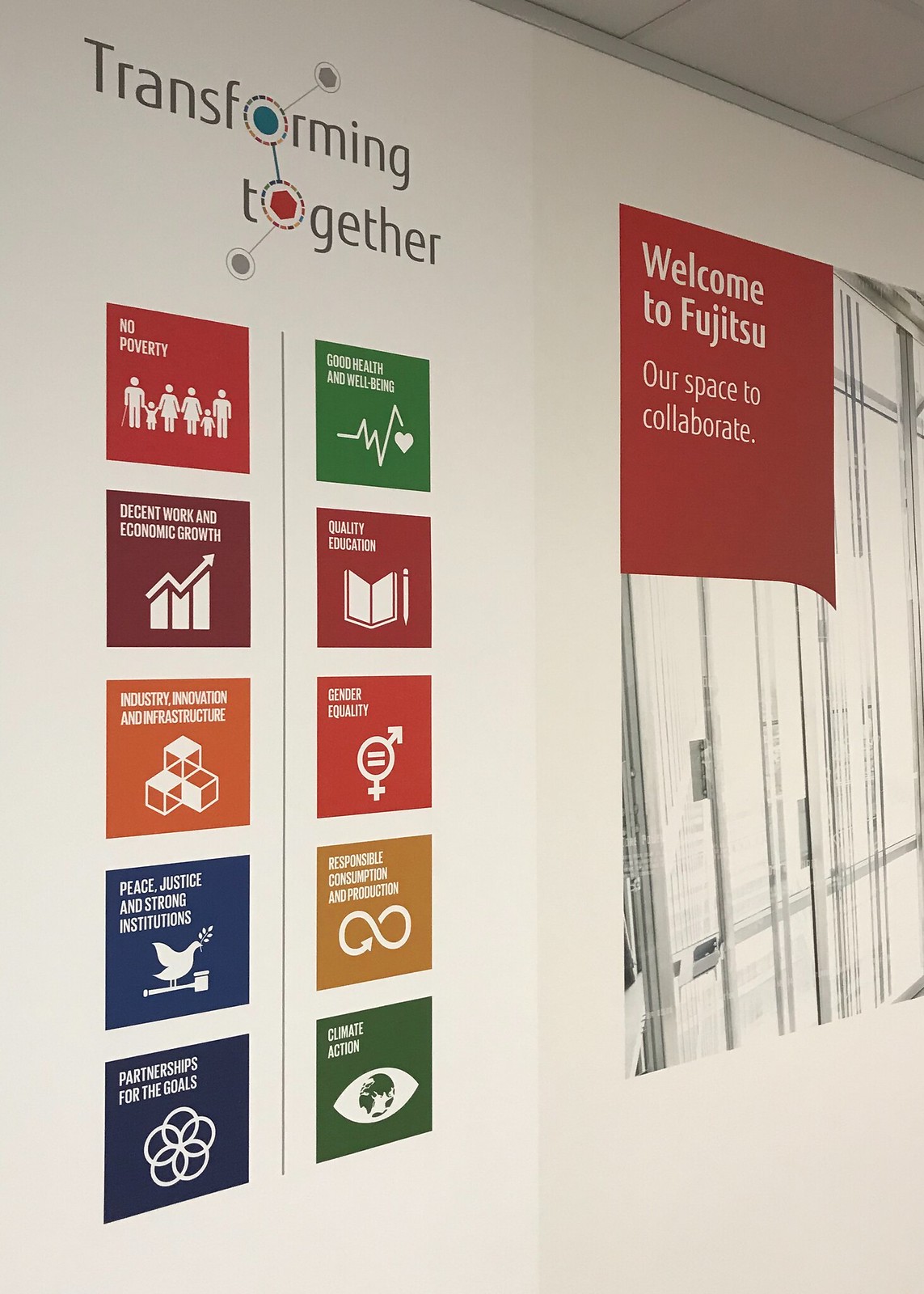This photograph captures a detailed infographic displayed at an angle, either on a wall or a projection screen, making it a bit challenging to see clearly. Dominating the graphic is the phrase "Transforming Together" against a white background. Below this, a series of brightly colored squares each feature a unique white graphic, alongside text depicting various initiatives and goals. These include themes such as "No Poverty," "Decent Work and Economic Growth," "Industry, Innovation and Infrastructure," "Peace, Justice, and Strong Institutions," "Partnerships for the Goals," "Good Health and Well-Being," "Quality Education," "Gender Equality," "Responsible Consumption and Production," and "Climate Action." Each icon within the squares visually represents these themes. To the right, there’s a larger red box with the inscription "Welcome to Fujitsu, Our Space to Collaborate," situated next to what appears to be a photograph of windows or glass doors. The image merges various social and corporate initiatives, highlighting a commitment to collaboration and sustainability, as emphasized by the repeated elements across multiple descriptions.